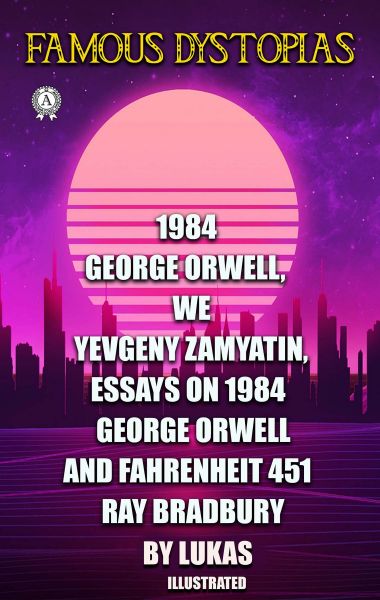This image appears to be a designed poster or book cover featuring a dystopian theme. Dominating the top in an ornate yellow font are the words "FAMOUS DYSTOPIAS," with a circular emblem or medal containing an "A" right beneath it. The background showcases a cityscape with silhouetted skyscrapers against a sky painted in shades of purple, dotted with stars. Central to the design is a fragmented, orange-ish moon. The grid-like ground comprises deep purple with lighter purple lines. The image lists various famous works of dystopian literature in white, all caps font, starting mid-way through the moon and continuing downwards: "1984, George Orwell, WE, Yevgeny Zamyatin, Essays on 1984, George Orwell, Fahrenheit 451, Ray Bradbury." The text concludes with "by Lucas" and a smaller "ILLUSTRATED" at the bottom. This graphic, which is neither a photograph nor a painting, appears to serve as an advertisement or cover for a collection of dystopian classics.